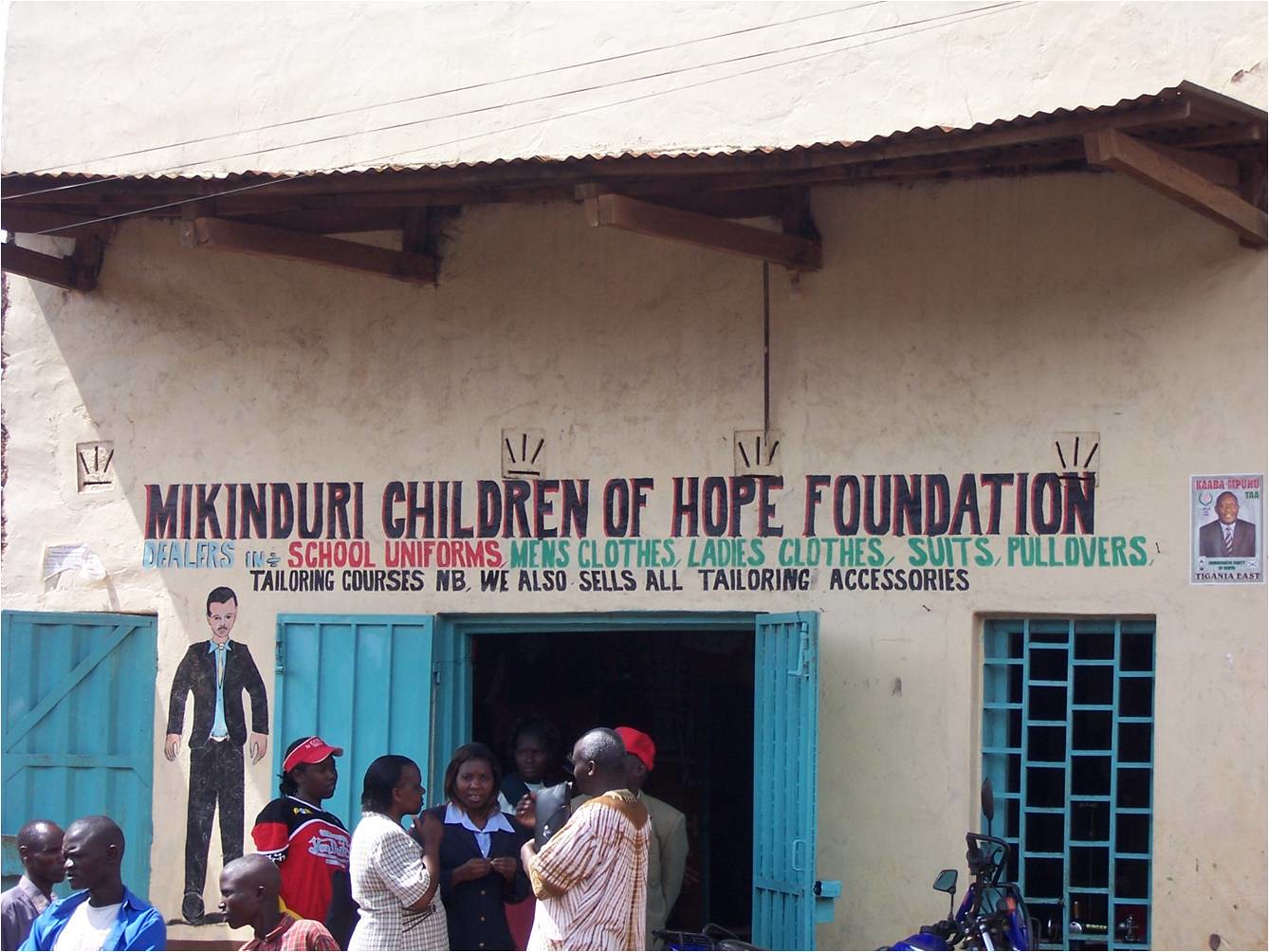In this image, a group of nine people, both men and women, are standing in front of a tan-colored building with a stone-like appearance and a beige paint job. The building features a pitched roof made of zinc, supported by brown wooden rafters holding up a tan awning. Prominently displayed on the building in bold lettering is "Mkhinduri Children of Hope Foundation." Below this, the sign advertises, "Dealers in school uniforms, men's clothing, ladies' clothes, suits, pullovers, tailoring courses, NB. We also sell all tailoring accessories." The structure includes bright blue double doors and blue-paned windows, which add a vibrant contrast to the beige exterior. Three power lines can be seen running in front of the store, which appears to be in a location outside of the United States, as indicated by the building's design and the presence of a predominantly Black community in the photo. The individuals are positioned directly in front of the blue double doors, engaged in conversation.